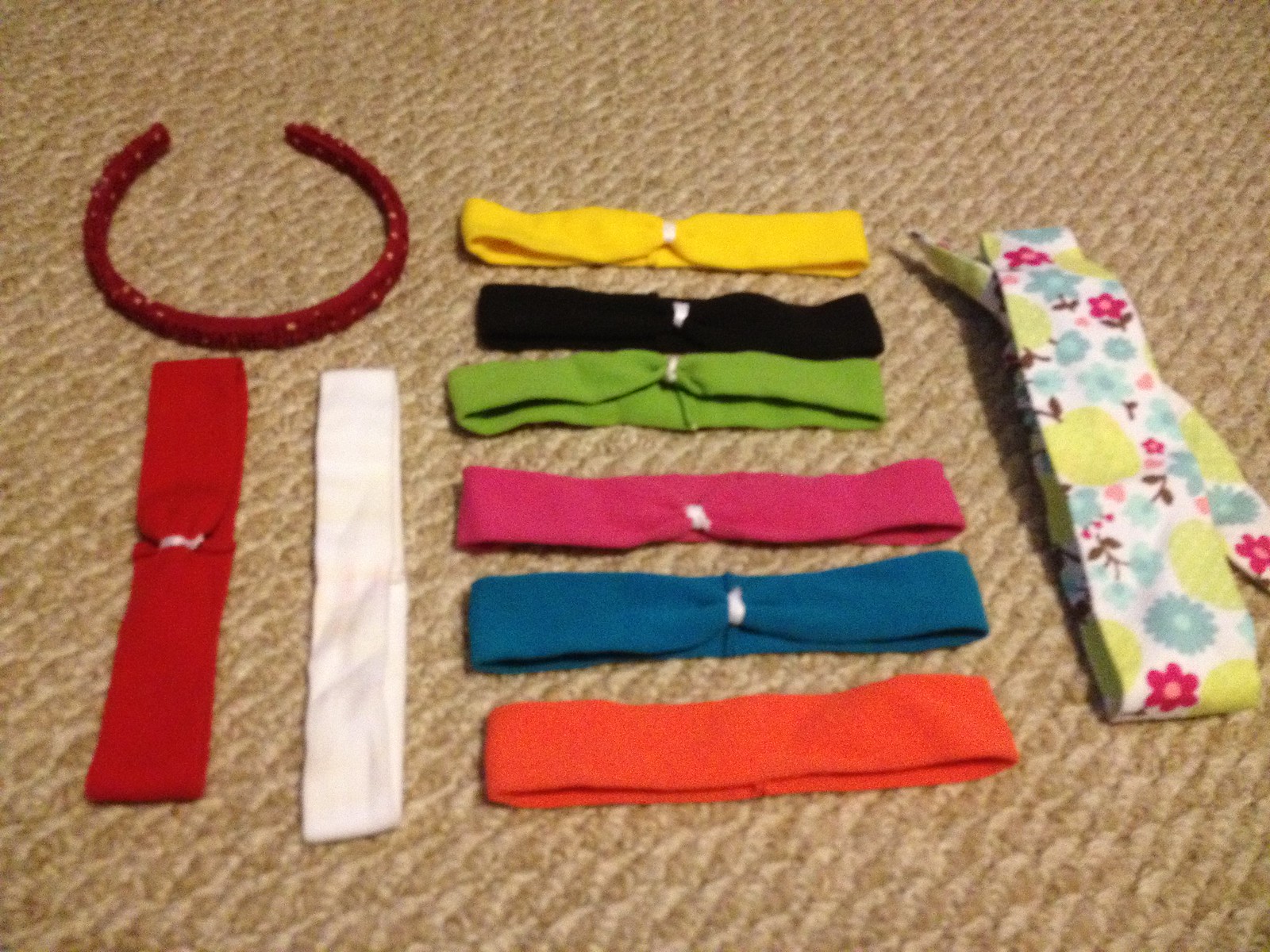This image features a collection of headbands displayed on a light brown, rugged oatmeal or beige Berber carpet, which appears slightly dirty and dimly lit, giving the photo a washed-out appearance. In the upper left corner, there's a solid, U-shaped plastic headband in red, resembling a bracelet but designed for a baby or a small child. Directly below it, there are two folded fabric headbands: one red and one white. Further to the top, there is a line of headbands in assorted colors arranged horizontally: yellow, black, green, pink, blue, and orange. Finally, on the far right, a white fabric headband adorned with a red, blue, and lime green flowery design completes the collection.